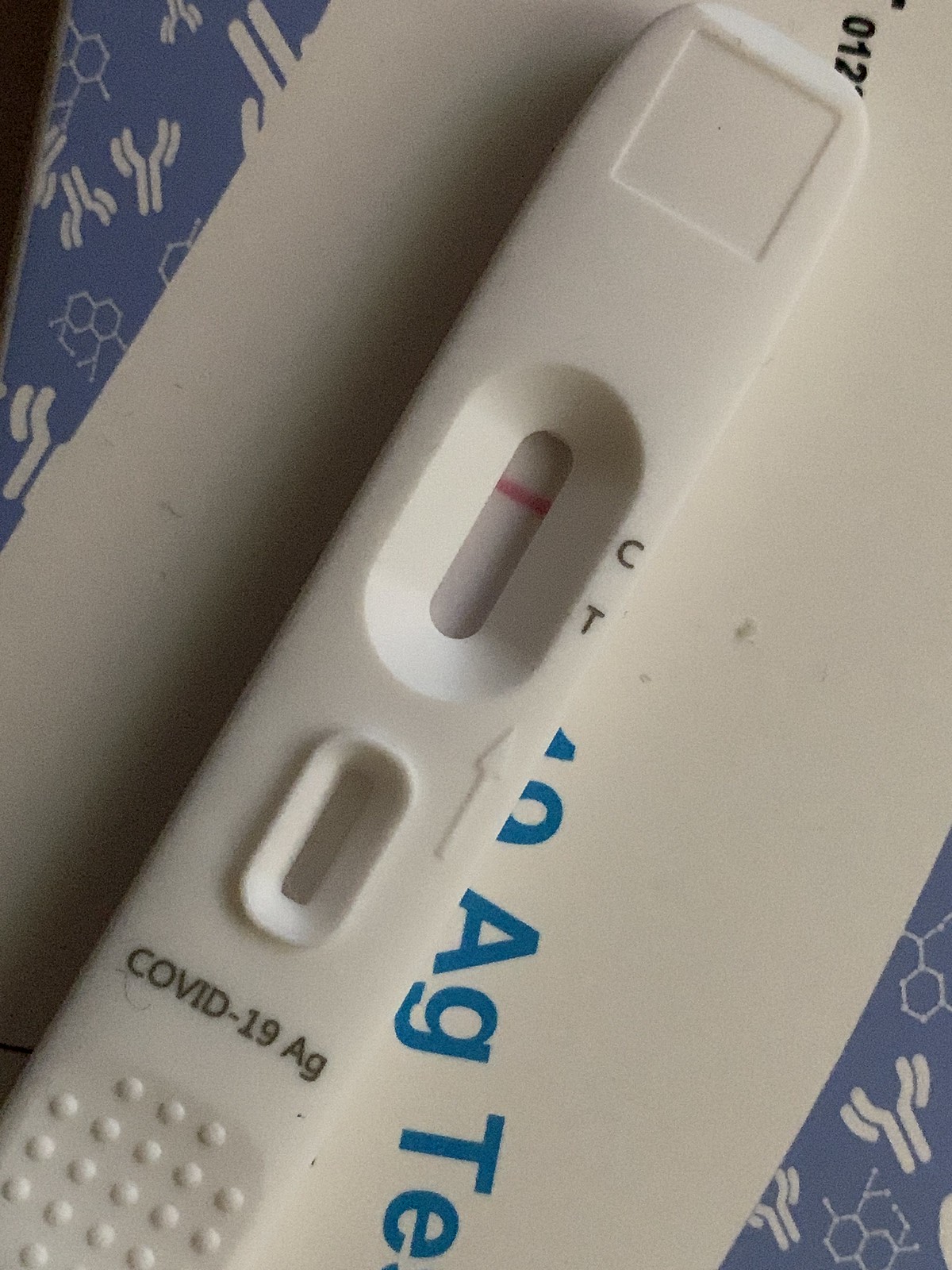In this detailed photograph, a close-up view of a COVID-19 rapid antigen test is prominently featured. The test consists of a long, white plastic tube, diagonally positioned on what appears to be a tablecloth. The tablecloth is light blue with intricate, abstract floral and plant designs. Beneath the test strip, a white package is partially visible, with lettering that includes "19," "AG," and "TE" indicating it's part of the test kit.

The COVID-19 test strip itself is marked at the bottom with small, raised dots, and just above them, bold black text reads "COVID-19 AG." Above this text are two window inserts; the larger one is highlighted with a small, red horizontal line indicating the test result. The overall composition of the photograph provides not only a clear view of the test but also an aesthetically pleasing background, emphasizing the importance and context of the rapid antigen test in a domestic setting.